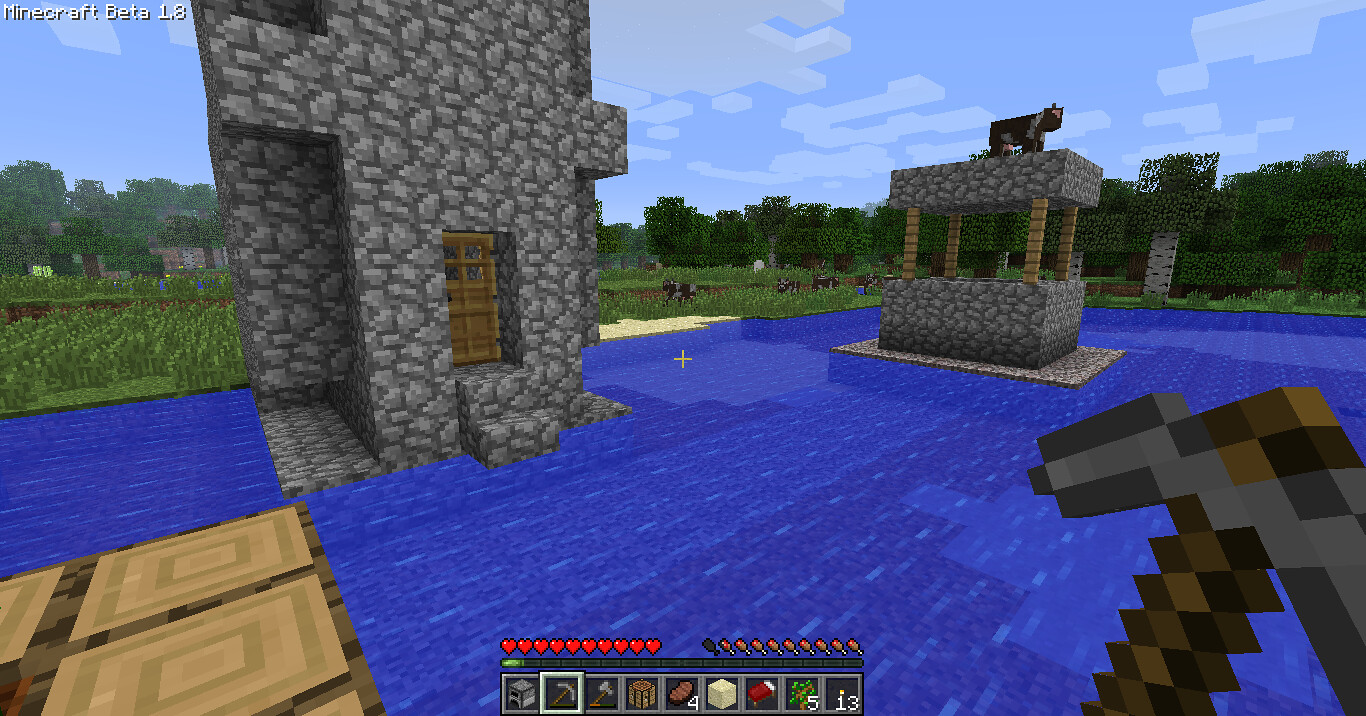This screenshot from the video game Minecraft showcases a large, creatively constructed pool. Two prominent stone structures are built along its edges. The first structure, positioned towards the center-left, is a tall stone building accessed by a small set of steps leading up to a brown door. In the bottom right corner of the image, a pixelated Minecraft axe or possibly a sword is visible. The second structure, located at the top right, is another stone formation topped with a cow. The background is teeming with pixelated grass, with various animals visible, and dotted with the iconic, blocky trees that define the Minecraft landscape.